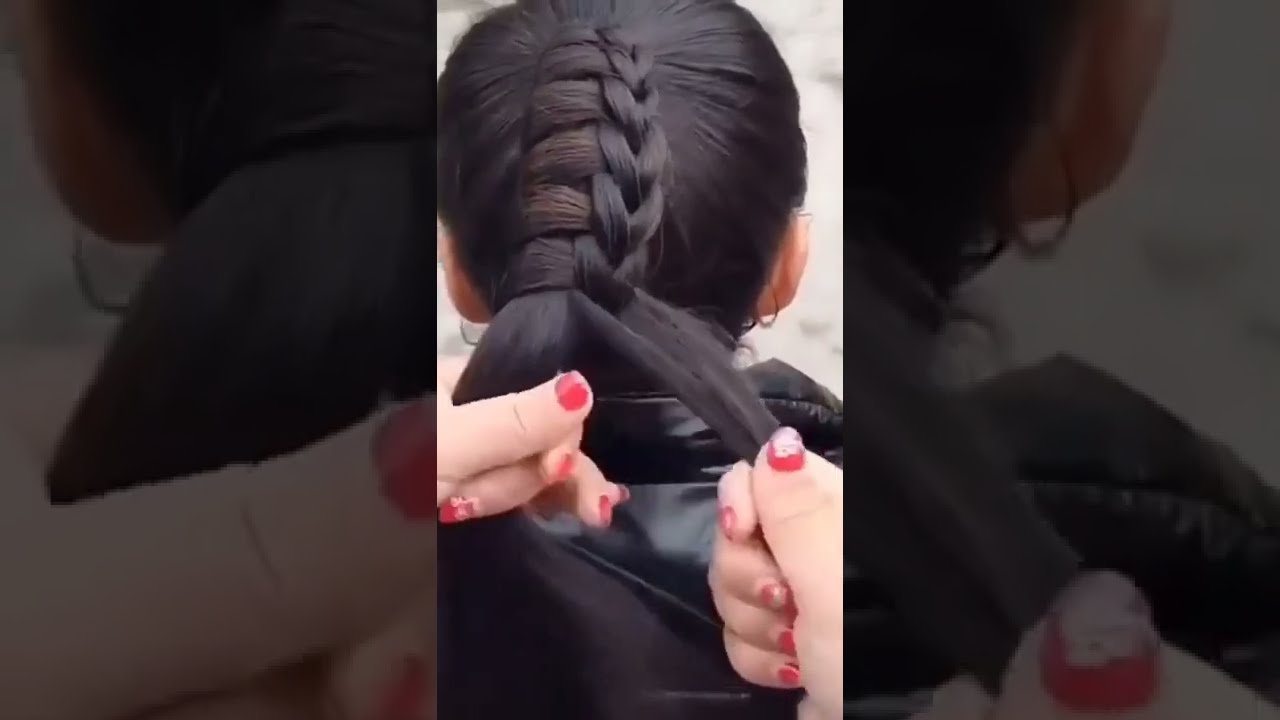The image is a close-up photograph of a woman with dark, shiny hair, as she gets her hair braided by another person. The scene is captured from a first-person perspective, focusing closely on the back of the woman's head and shoulders, revealing her black leather puffer jacket with a collar. Her hair is styled in a ponytail that is being intricately braided down the right side of her head. The braider's hands, adorned with short red fingernails with white designs, are prominently positioned behind the woman's shoulders, holding two strands of hair. The composition features a grayscale, blown-up background that frames the central image, emphasizing the action. The background is blurred, showing off-white and grayish tones, suggesting an outdoor setting, possibly on a sidewalk or pavement. Slightly visible are details such as possible earrings or curled hair strands near the woman’s ears, adding a touch of intricacy to the overall image.